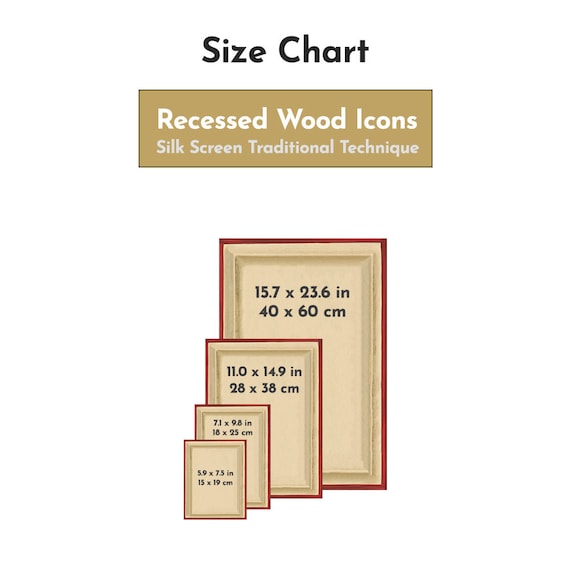The image displays a detailed digital rendering of a size chart for recessed wood icons, employing a traditional silkscreen technique. At the top, the chart is labeled "Size Chart," with text in white on a tan background reading "Recessed Wood Icons" and "Silkscreen Traditional Technique." Below this, the chart features a series of four tan rectangles, each framed by a bright red outline, arranged from largest to smallest. The dimensions for each rectangle are provided in both inches and centimeters. The largest rectangle measures 15.7 by 23.6 inches (40 by 60 centimeters), followed by the next at 11.0 by 14.9 inches (28 by 38 centimeters), then 7.1 by 9.8 inches (18 by 25 centimeters), and the smallest at 5.9 by 7.5 inches (15 by 19 centimeters). The background remains white, enhancing the clarity and visibility of the outlined frames and their corresponding sizes.